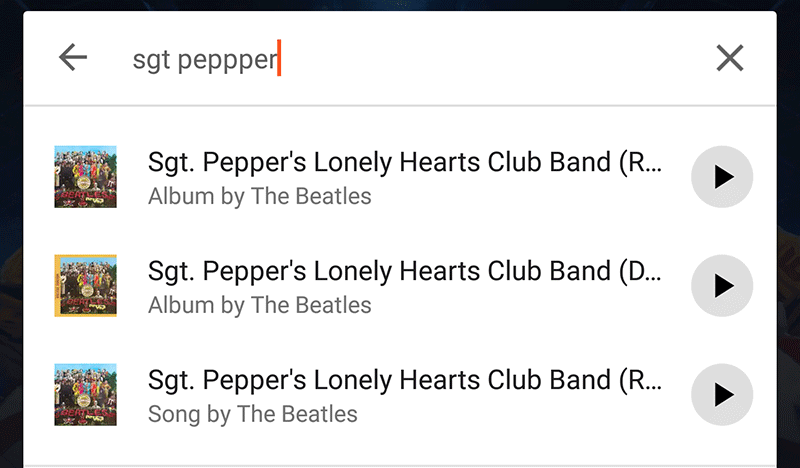The image is a screenshot of a search interface where the user appears to have looked up "SGT Pepper." On the right side of the search bar, there is an 'X' button for clearing the search query, and on the left side, there is a back arrow pointing to the left, presumably for navigating to the previous page. Below the search bar, three nearly identical search results are displayed. The first result reads "SGT Pepper's Lonely Hearts Club Band," followed by "(R" with the remainder of the text cut off. The second result is identical except for the distinction at the very end, where it reads "(D" before being truncated. The third result aligns with the first, indicating they might be different versions or formats of the same album. To the right of each search result, a play button is visible, suggesting that the user can play the selected item directly from the search results.